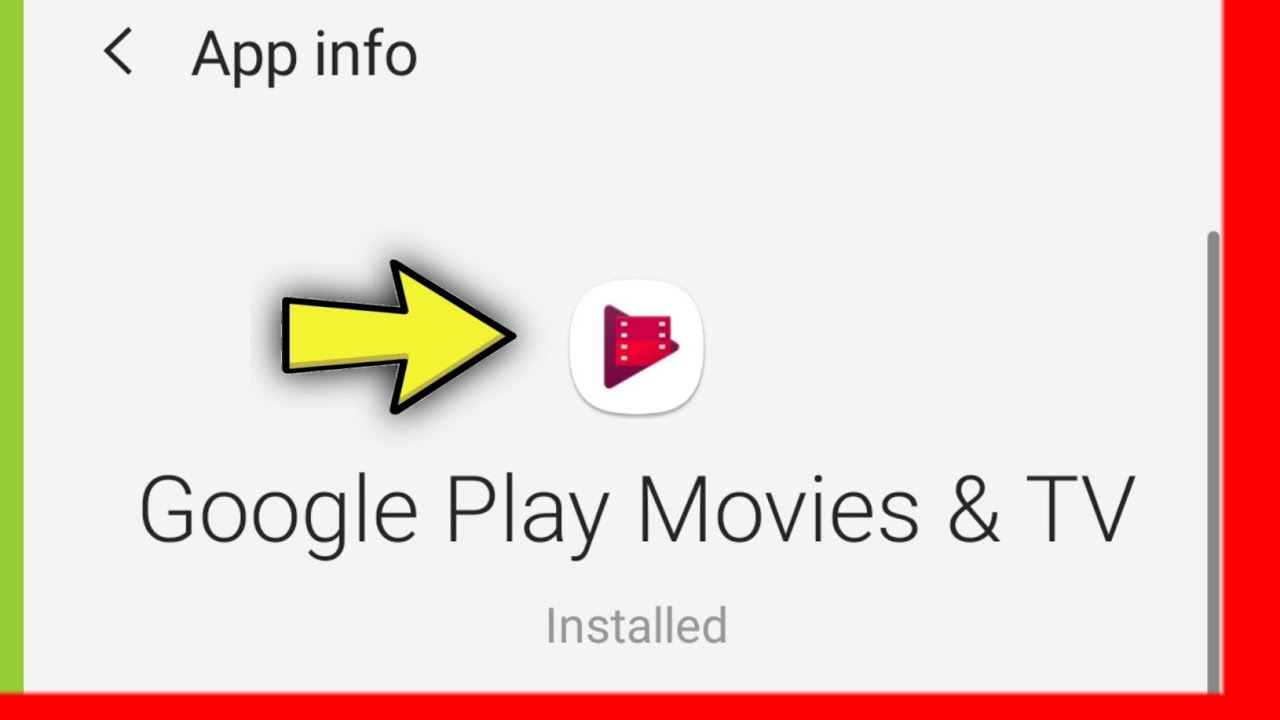This image is a promotional graphic for Google Play Movies and TV, formatted as a horizontal rectangle. A prominent red bar lines the right edge, transitioning into the bottom edge. Adjacent to this red bar on the right, there is a gray line running vertically but stopping short before reaching the top. On the left edge, a green bar extends upwards, stopping right above the red bar at the bottom. The main background is light gray, with text appearing in either gray or black. 

In the upper left corner, a left-pointing caret symbol in black accompanies the black text "App Info." Central to the image is the icon for Google Play Movies and TV, represented as a rounded square button. This button features a maroon play button with a right-pointing triangle overlaid by an icon resembling a film strip. Highlighting this icon is a large yellow arrow outlined in black. Beneath the app icon, the text "Google Play Movies and TV" is prominently displayed in black, with the word "installed" appearing below it in gray.